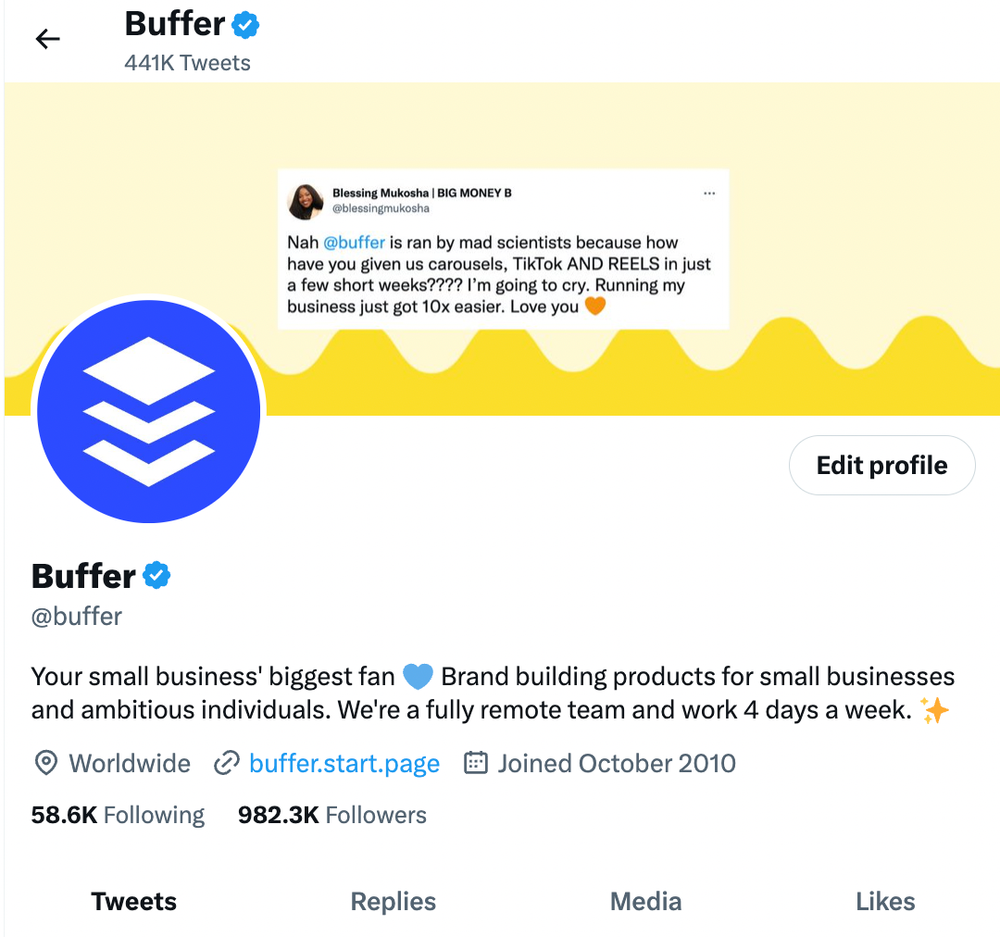Buffer's official Twitter profile features a distinctive layout. At the top, "Buffer" is displayed prominently in black capital letters with a blue verification tick next to it, accompanied by the text indicating they have made 441,000 tweets. The banner background is light yellow, decorated with a stylized darker yellow mountain range at the bottom.

The profile picture is a blue circle with a white diamond at the top and two arrow-like shapes underneath, which mimic the diamond's shape without being complete diamonds. Positioned in the middle of the banner is a tweet from Blessing Mokosha, praising Buffer for their updates: "Big money be nah at Buffer is a ran by mad scientists because how have you given us carousels tik-tok and reels in just a few short weeks I'm gonna cry I'm going to cry running my business just got ten times easier love you," accompanied by an orange heart. Her profile picture shows a smiling Black woman with long hair.

Buffer's description reads: "Your small business's biggest fan 💙 Brand building products for small businesses and ambitious individuals. We're a fully remote team and work four days a week." Beside this, there is an orange star emoji.

The statistics for Buffer's account display that they are following 58.6 thousand other accounts and have amassed 982.3 thousand followers.